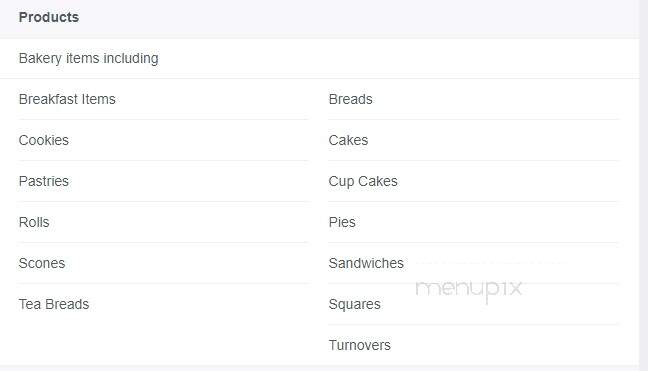The image features a menu with a light grey horizontal bar running across the top and a thin grey vertical bar descending along the right-hand side. In the top-left corner, "Products" is written in black font. Below this, a list of bakery items is presented on the left-hand side, including breakfast items, cookies, pastries, rolls, scones, and tea breads. On the right-hand side, starting somewhat lower than the list on the left, are additional products: breads, cakes, cupcakes, pies, sandwiches, squares, and turnovers. A light grey watermark reading "MENUP IX" or possibly "MENUP 1X" is faintly visible between the "sandwiches" and "squares" listings.